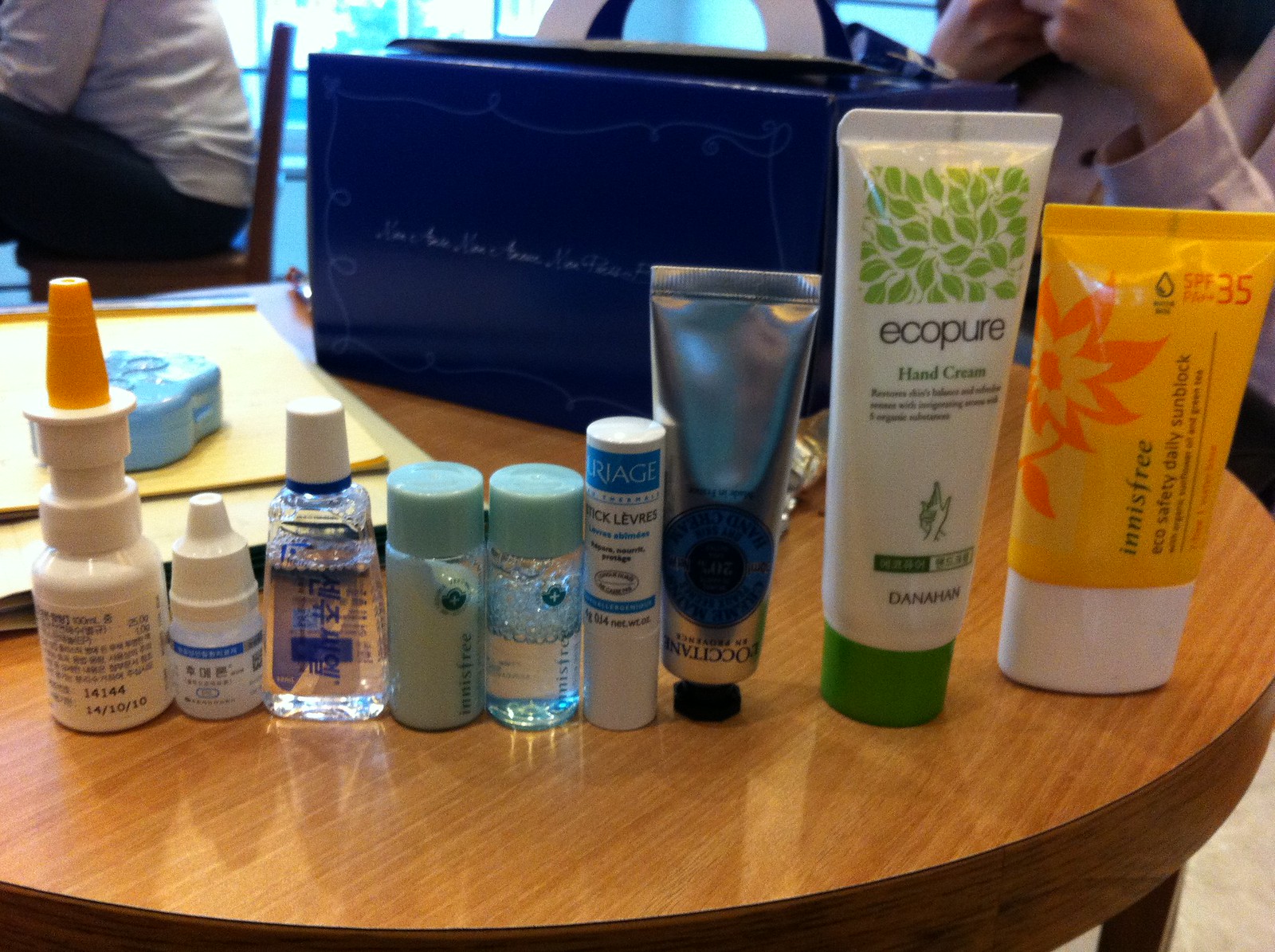In this detailed indoor scene, various personal care and medicinal items are arranged on a counter or table. Among these items:

- A notable yellow lotion tube adorned with an orange flower, highlighted for its moisturizing properties and SPF 35 sun protection with water resistance, as indicated by a water droplet icon.
- Next to the lotion, a white tube with green leaves and a green lid labeled "Eco Pure Hand Cream" showcases its natural essence.
- A blue tube with an unreadable label, featuring a silver end, adds a contrasting touch to the array.
- A blue and white chapstick lies nearby, compact and handy.
- Two bottles with aqua-colored lids and bluish-green glass suggest cleaning solutions.
- Positioned beside these, a hand sanitizer ensures cleanliness.
- A bottle of eye drops stands ready, addressing vision needs.
- An orange-tipped antihistamine injector, reminiscent of medical precision, complements this collection alongside a nondescript white bottle.

In the background, a blue bag catches the eye, partially obscuring an individual in a white shirt whose identity is indistinguishable due to the angle. This cohesive display of everyday essentials captures a snapshot of readiness and care.